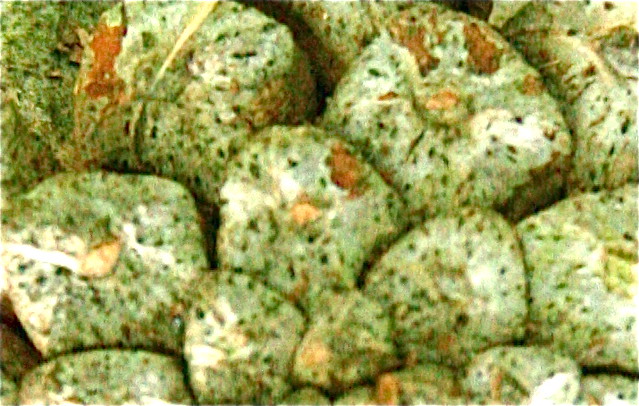The image is a low-quality, grainy, and blurry photograph likely taken with a night vision filter. It depicts a collection of rounded, irregularly shaped objects that appear somewhat disgusting and are greenish with white on top, interspersed with orange patches. The objects resemble moldy marshmallows or perhaps birds with spotted feathers, clustered together in a somewhat squished, connected manner. The picture shows a vaguely structured arrangement: about five objects in the front row, with successive rows displaying objects in decreasing numbers—five, four, and three, respectively. The upper left corner is predominantly green, possibly indicating foliage or grass, contributing to the overall uncertain and cluttered visual presentation. Shadows, black spots, and some indications of knots or protrusions add to the indistinct and confused scene.